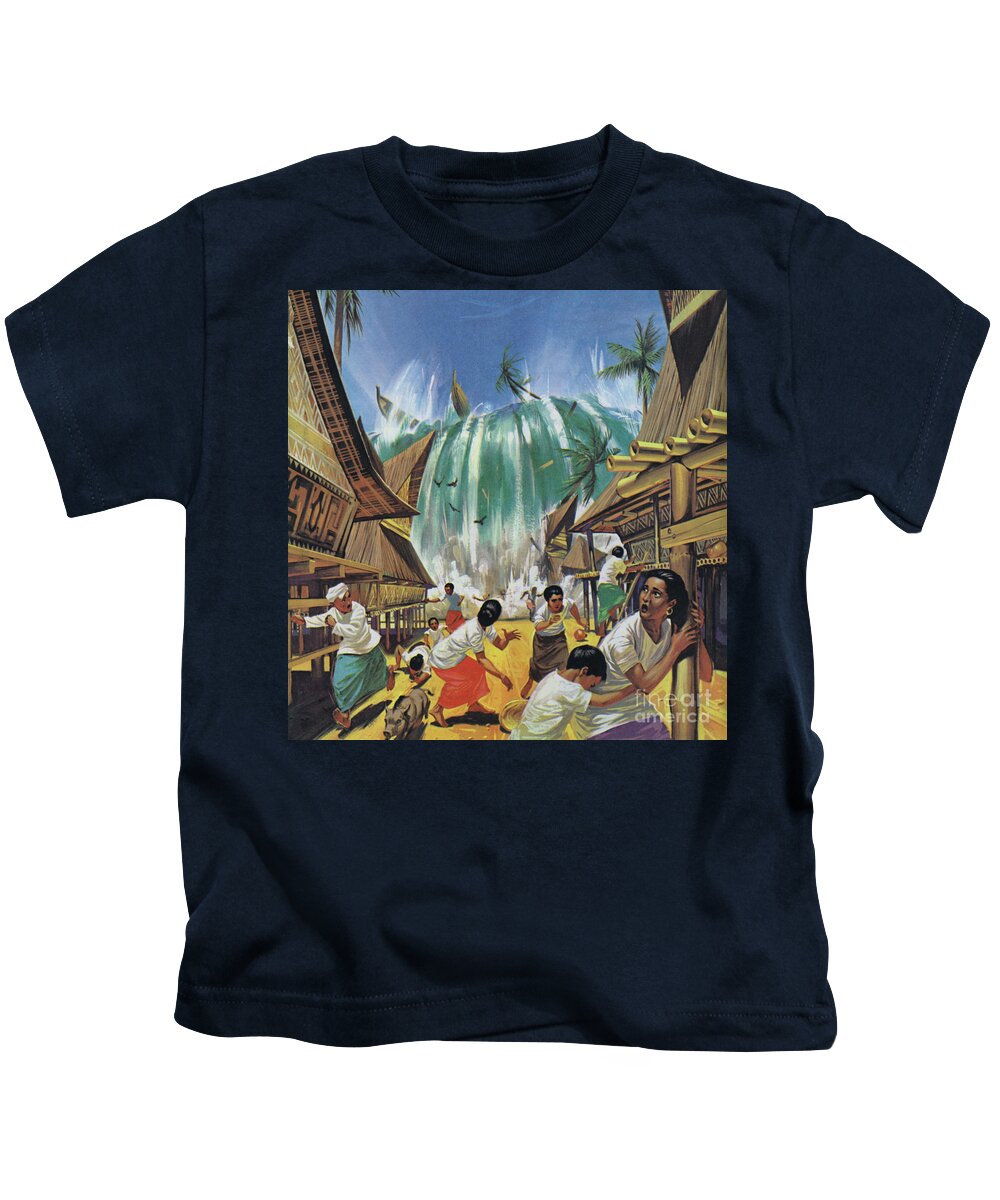The image features a dark-colored, short-sleeved, crew-neck t-shirt displayed against a plain white background. The t-shirt prominently showcases a detailed square print on the front. The print vividly depicts a dramatic scene of a coastal village being overwhelmed by a massive dark greenish wave, suggestive of a tsunami. This wave is depicted with elements like sailboats, surfboards, trees, and palm trees being swept away. In the foreground, villagers with light brown skin, black hair, and wearing traditional attire, such as skirts and a man with a white turban, are seen running for their lives along a sandy, light brown street. The scene is framed by dark brown buildings with bamboo and straw roofs on both sides. A woman clutching a pole with a child beside her, amidst other panicked villagers, is also visible. Above the chaotic scene, the sky is a calm blue. The illustration is captioned with "Fine Art America" in the bottom right corner.